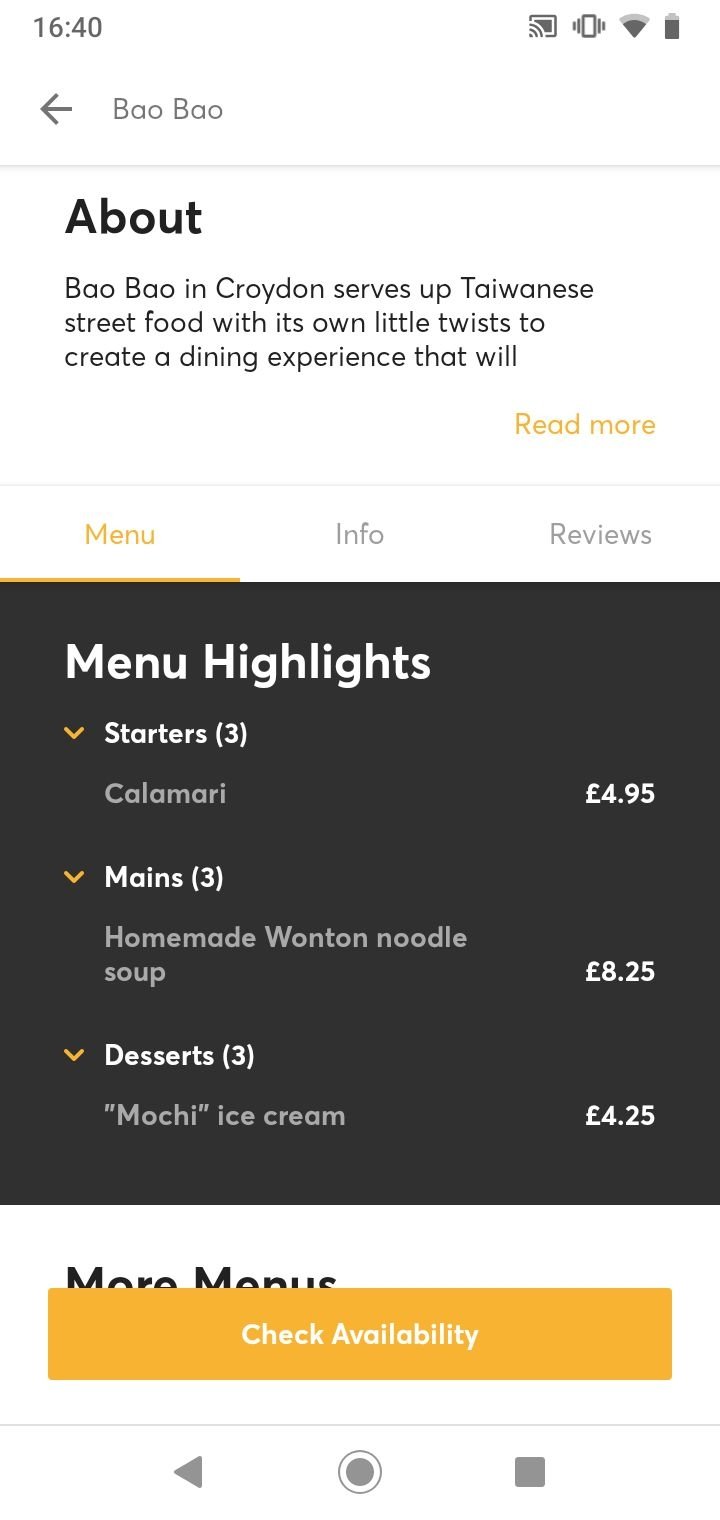This screenshot depicts the interface of a website. At the top right corner, the time is displayed as 16:40 (4:40 PM), accompanied by symbols for Wi-Fi and battery levels. Below this, there is a navigation bar with a left-facing arrow and the text “Bao Bao.” Underneath, the phrase "Bao Bao in Croydon serves up Taiwanese street food with its own little twists to create a dining experience that will..." appears, followed by a "Read more" link highlighted in yellow, indicating a clickable link.

The next line features three menu options: "Menu," "Info," and "Reviews," with "Menu" highlighted in yellow, indicating it is the currently selected option. Below this is a black box with the heading "Menu Highlights." Within the box, three sections of the menu are displayed:

- **Starters**: Calamari, priced at £4.95.
- **Mains**: Homemade Wonton Noodle Soup, priced at £8.25.
- **Desserts**: Mochi Ice Cream, priced at £4.25.

Beneath these listings, another heading is partially obscured by a yellowish-orange bar with the text "Check Availability."

At the very bottom of the screenshot, there are navigation icons: a right-facing arrow, a circle within a circle, and a square.